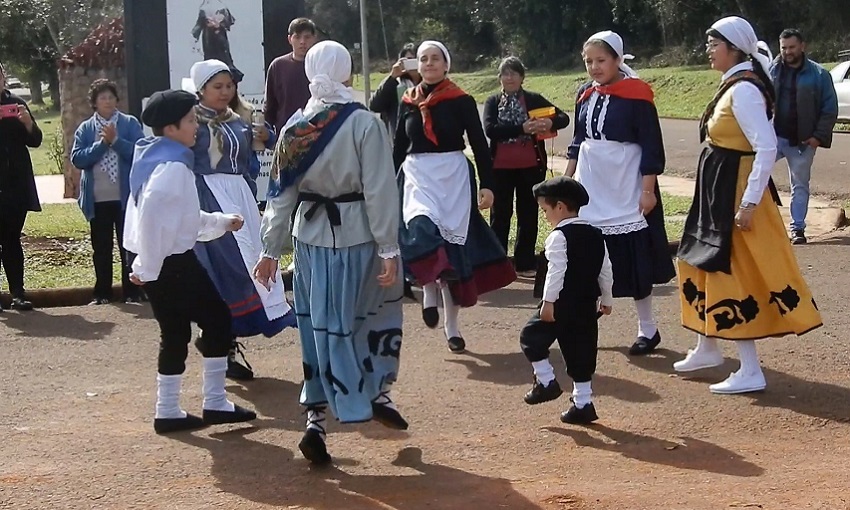In this daytime photograph, a group of people is seen dancing in a circle on a beige gravel surface, likely within a park area. The participants, seemingly in a traditional cultural setting, feature five women and a young girl accompanied by two boys. The women are dressed in long modest dresses with white bandannas and aprons, and most are in black shoes except one in white shoes. Their attire is varied, including two in black dresses, two in blue dresses, and one in a yellow dress with a black apron. Thick white socks complement their outfits.

The two boys, one approximately three and the other around nine, are wearing traditional attire, including black trousers tucked into thick white socks, white shirts, scarves, and black berets (tams). Their black shoes match the rest of their attire, exuding a cultural charm.

Spectators in casual jackets, hinting it might be cool, are observing the performance. In the background, a grassy lawn transitions to a line of trees, completing the park setting. A banner with an image potentially depicting a nun dressed in a black gown with a white neckband is also visible, adding an intriguing element to the scene. The overall atmosphere is bright and sunny, illuminating the traditional dance and vibrant costumes of the participants.